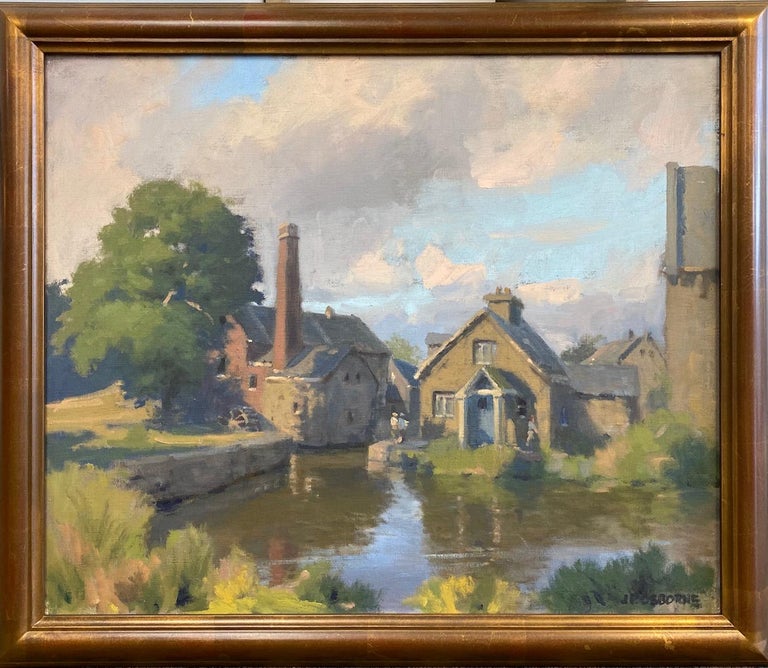This photograph showcases a painting of a serene countryside village, enhanced for online listings with a solid white background. The painting is encased in a well-worn brown frame, replete with marks and nicks lending it an antique look. Centrally depicted is a peaceful small town consisting of light gray stone buildings and houses. Noteworthy structures include a prominent building on the right with a tall stone tower, which resembles a grain silo, and another on the left featuring a large water wheel partially visible amongst the foliage. This wheel connects to a river or pond that meanders from the lower left corner across to the right, bordered by a stone wall and lush greenery. In the distance and toward the middle, a reddish-brown chimney stands out against the overcast sky dominated by grayish-white clouds, with patches of blue peeking through. The intricate details of the town and the tranquil reflections in the still water culminate in a calming landscape that captures the essence of rural life.